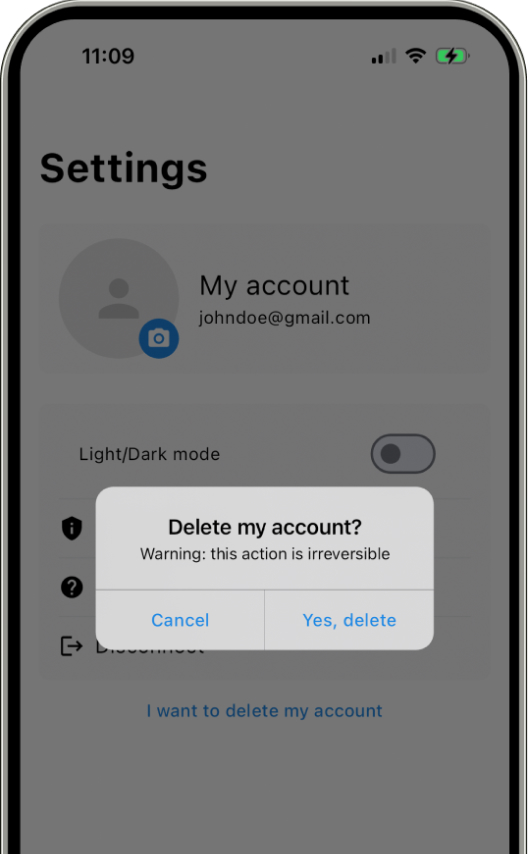The image presents a mock-up of a smartphone interface, specifically focusing on the option to delete a Gmail account. The smartphone showcased has distinct curved bevels, black borders, and a silver frame. The sides of the phone are devoid of any visible buttons, emphasizing its sleek design. The screen displays at 11:09 with two signal bars, full Wi-Fi connectivity, and a nearly full battery indicator.

On the screen, the settings menu is open, featuring a generic profile image and the account information for "John Doe" (john.doe@gmail.com). Options present include the ability to change the profile picture, toggle between light and dark modes, and various security settings. 

A prominent white pop-up window overlays the screen, displaying a warning message: "Delete my account. Warning: this action is irreversible." Below this message, a thin gray horizontal bar and a vertical divider organize two interactive choices: "Cancel" in blue text on the left, and "Yes, delete" on the right. At the bottom of the grayed-out background, blue text states, "I want to delete my account," indicating that the user has already engaged this function, leading to the appearance of the pop-up.

Approximately 70% of the phone is visible in the image, with the bottom portion cut off, focusing solely on the relevant interface features without unnecessary visual elements.